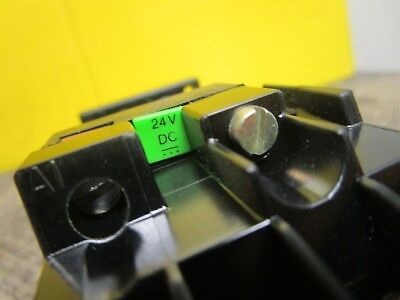This close-up photograph captures a section of unidentified, metallic equipment, primarily composed of dark gray, shiny material. Central to the image is a green tag prominently displaying "24VDC," indicative of a 24-volt direct current electrical component. Adjacent to this tag is a silver-colored set screw with a slot head. Printed or embossed on the left-hand side, there is a marking that reads "AI" or "A1." The background contrasts vividly with a bright, cheerful yellow, although it remains out of focus. Despite the detailed elements, the precise nature of the equipment depicted remains unclear.